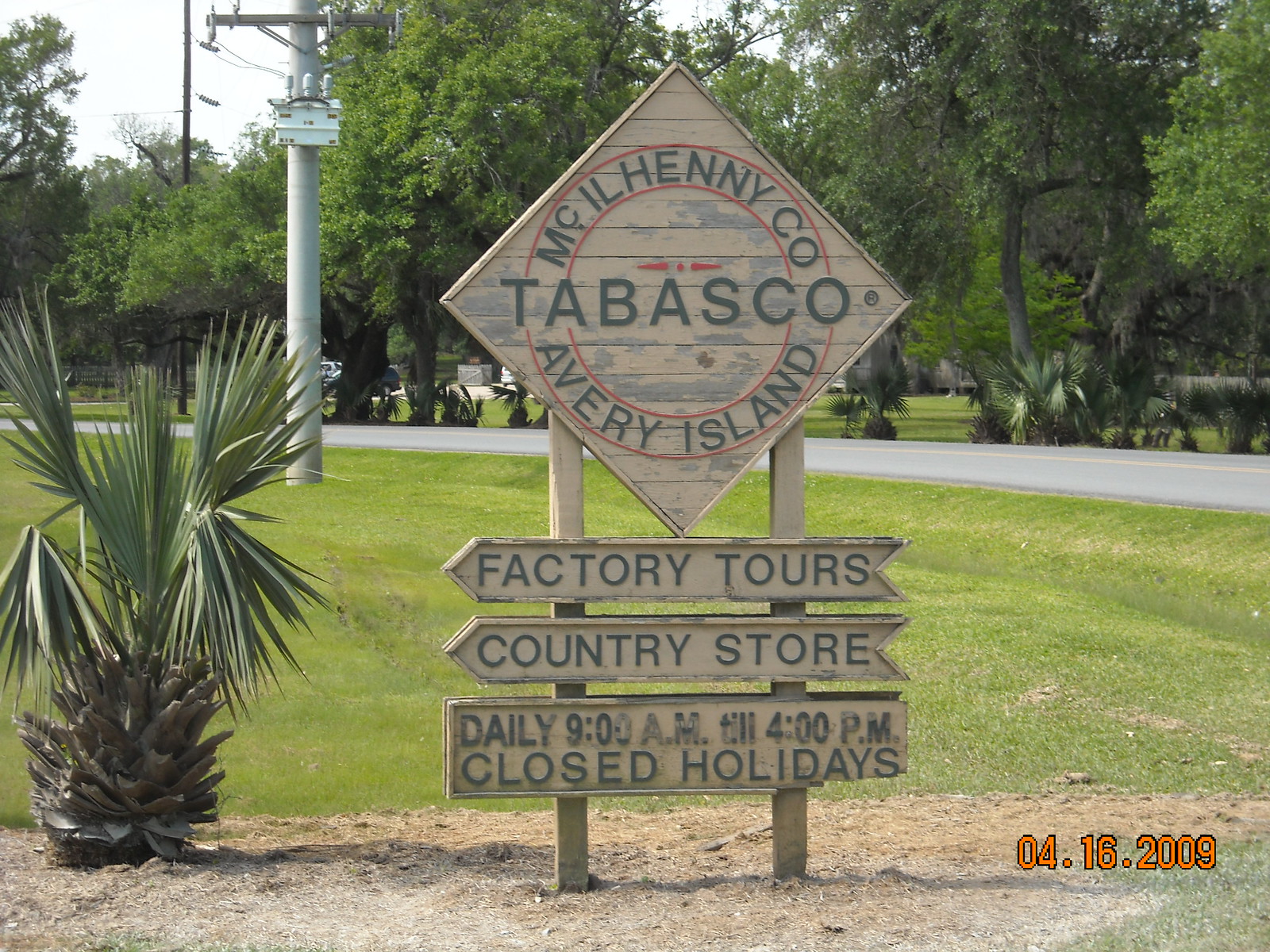This photograph, rectangular in shape, depicts a wooden sign standing in a grassy area with a patch of dead, brown grass directly beneath it. To the left of the sign is a plant with spiky green leaves. The background reveals a two-lane road flanked by more green grass, a telephone pole with wires, and a dense cluster of trees further off. The sign itself is supported by two wooden posts and features a diamond-shaped top section with a red circle in the middle. Around the circle, it reads “McIlhenny Company” above and “Avery Island” below, while “Tabasco” is prominently displayed across the center in gray letters. Beneath this diamond, there are two horizontal arrow-shaped slats pointing to the left, marked “Factory Tours” and “Country Store,” and a rectangular sign at the bottom stating, “Daily 9 a.m. to 4 p.m. Closed Holidays.” In the lower right-hand corner of the photo, the date "04.16.2009" is printed in orange.